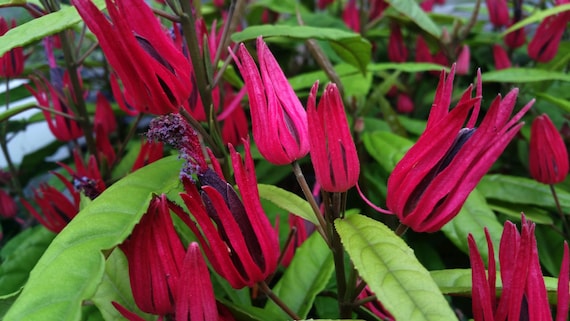This image captures a vibrant and colorful flowering plant with rich magenta blossoms and bright green, slender leaves. The flowers, which feature both pink and deep purple shades, extend upwards and outwards, resembling hands grasping something with their pointed formations. Each blossom has a dark purple or violet pistil in the center, surrounded by tightly packed petals that appear oblong and vertical. Supporting these magnificent flowers are dark brown stems, adding a contrasting element to the overall composition. The background hints at the presence of water, enhancing the vivid and dynamic nature of the scene.